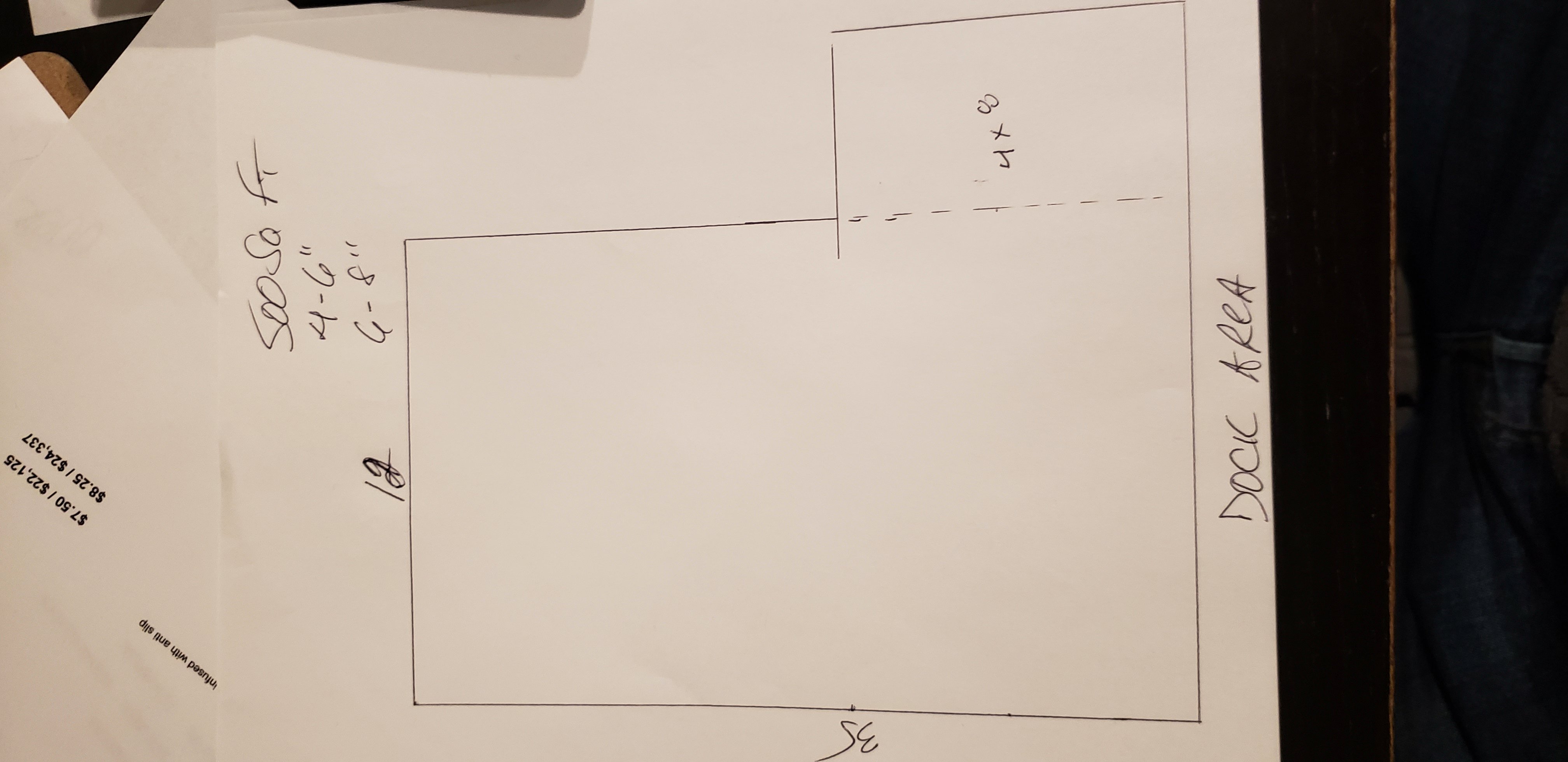This is an overhead image depicting a white piece of paper featuring a rudimentary architectural outline of a building space. The sketch is a rectangular shape with an additional wedge extension on the top right side. On the right side of the paper, near the building outline, there's a handwritten note labeled "door area." The dimensions of the layout are noted with the bottom edge measuring 32 feet, the right side 12 feet, and the wedge section is identified as 4 by 8 feet.

Additional text is present on the left side of the paper specifying "500 square feet," and measurements of "4 to 6 inches" and "6 to 8 inches." Beneath this main sheet, another piece of paper extends out slightly, showing what appears to be prices written upside down. The visible prices include "$7.50," repeated twice, and "$8.26." These details provide insight into both the spatial dimensions and potential costs associated with the outlined building space.